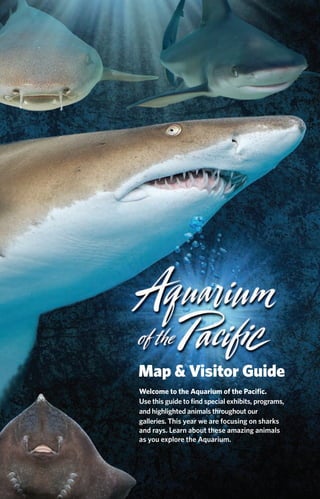This vibrant poster, likely the cover of a map and visitor guide for the Aquarium of the Pacific, showcases a striking underwater scene. Dominated by a dark blue background, the composition features multiple prominent sea creatures. At the center, a large shark with a brown body and white underbelly stretches horizontally, its crescent-shaped mouth brimming with sharp teeth aimed at the viewer. Above this central figure, two more sharks swim towards the observer, illuminated by beams of light from behind. In the bottom left corner, the underside of a flat stingray is visible, displaying its gills and mouth. Written in elegant white script at the bottom right, “Aquarium of the Pacific” is prominently displayed, followed by “Map and Visitor Guide” in smaller black text and a welcoming message. The text invites visitors to use the guide to explore special exhibits, programs, and highlighted animals, emphasizing the aquarium's focus on sharks and rays this year.